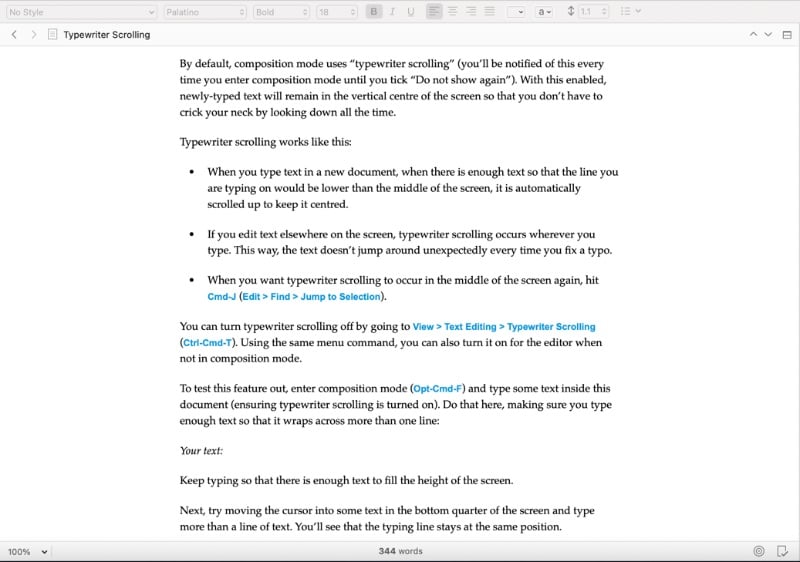This screenshot taken from a computer or laptop monitor showcases a word processing application, likely similar to Microsoft Word. The absence of a program title or identifiable icon makes it challenging to pinpoint the exact application. 

At the top of the interface is a light gray bar featuring several dropdown menus on the left. The first dropdown displays "No Style," the second reads "Palatina," and the third shows "Bold." Following these dropdowns is the traditional word processing formatting toolbar, which includes options for bold, indent, underline, left justify, center, right justify, and remove indentations, among others.

Below this, there are back and forward navigational arrows, a small piece of paper icon, and a label in bold black text reading "Typewriter Scrolling."

The main body of text begins with a bold paragraph stating: "By default, composition mode uses typewriter scrolling. You'll be notified of this every time you enter composition mode until you tick do not show again. With this enabled, newly typed text will remain in the vertical center of the screen so that you don't have to crick your neck by looking down all the time." This is followed by three bulleted points providing further instructions on using the typewriter scrolling feature. The final bullet point notes: "When you want typewriter scrolling to occur in the middle of the screen again, hit Command J, Edit, Find, Jump to Selection."

Additional features of the typewriter scrolling option are described further down. The last instruction in the text reads: "Next, try moving the cursor into some text in the bottom quarter of the screen and type more than a line of text. You'll see that typing line stays at the same position."

At the bottom left of the screen is a gray bar indicating "100%" with a dropdown arrow next to it. In the center, the text "344 words" appears in black, and on the far right, there is a bullseye-like circle icon followed by a gray outline piece of paper with a checkmark.